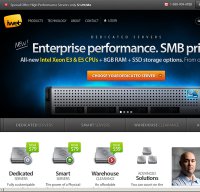The image features a white background with "Enterprise Performance SMB" prominently displayed, indicating a new release accompanied by an explanation. An orange rectangle filled with multiple lines of white text provides additional detailed information. There are four smaller images included: the first one focuses on smart warehouse solutions, packed with relevant details. Additionally, there is a photograph of a man with a shaved head, wearing a blue collared shirt, standing against a gray brick wall. At the bottom of the image, a gray scroll bar is visible.